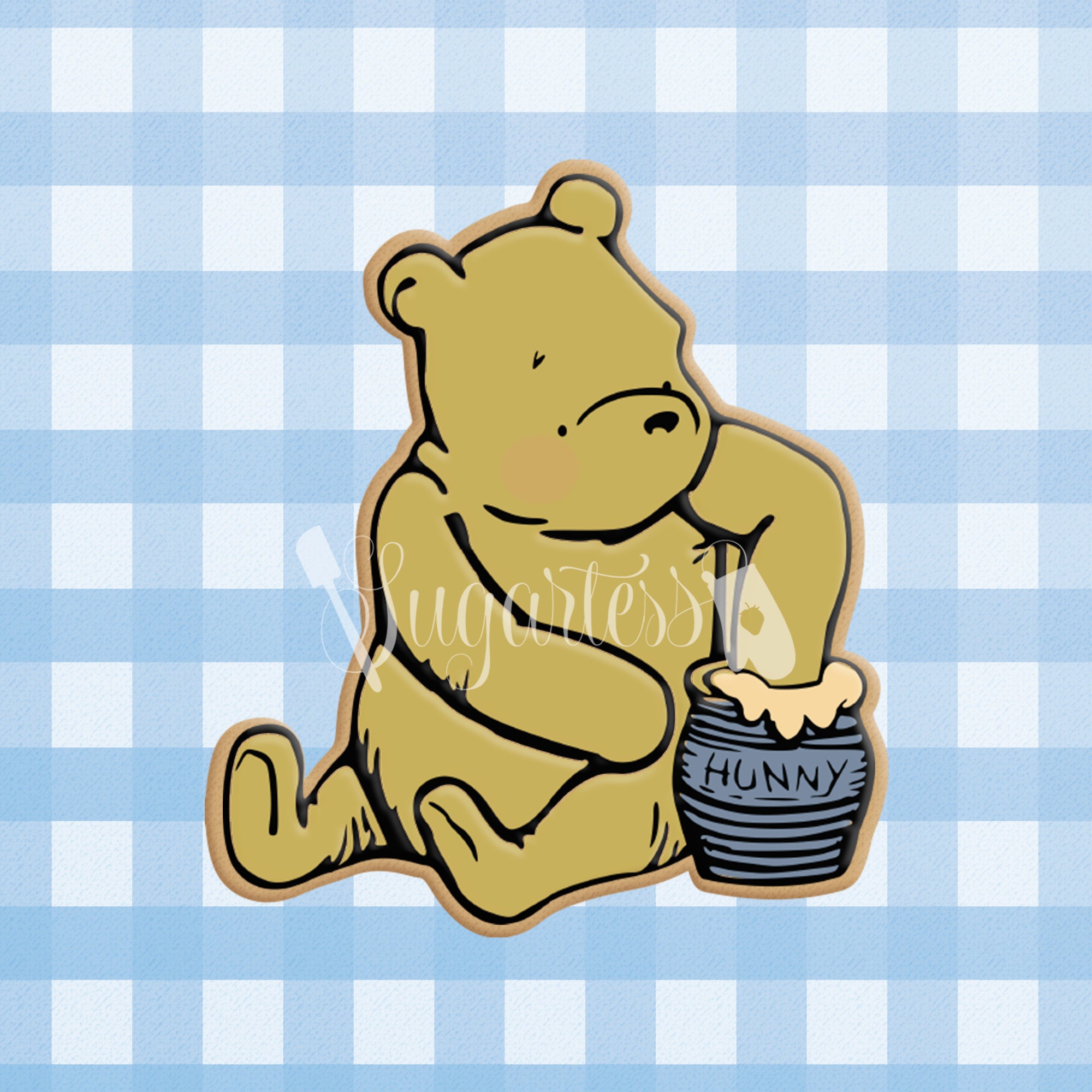The image depicts a caricature of Winnie the Pooh, sitting down on a checkered picnic blanket with light blue and white squares. Pooh, a yellow bear outlined in gold, has black button eyes and a frowning face as he focuses on a blue honeypot by his side. His left paw is dipped into the honeypot, which has black text spelling "HUNNY" and some honey oozing out from the top. The pot features black lines and white stripes. An additional element in the image is the faint text "SUGARLESS" appearing as a watermark script across Pooh’s chest. Overall, the scene captures Pooh's familiar honey-dipping moment against the classic picnic backdrop.